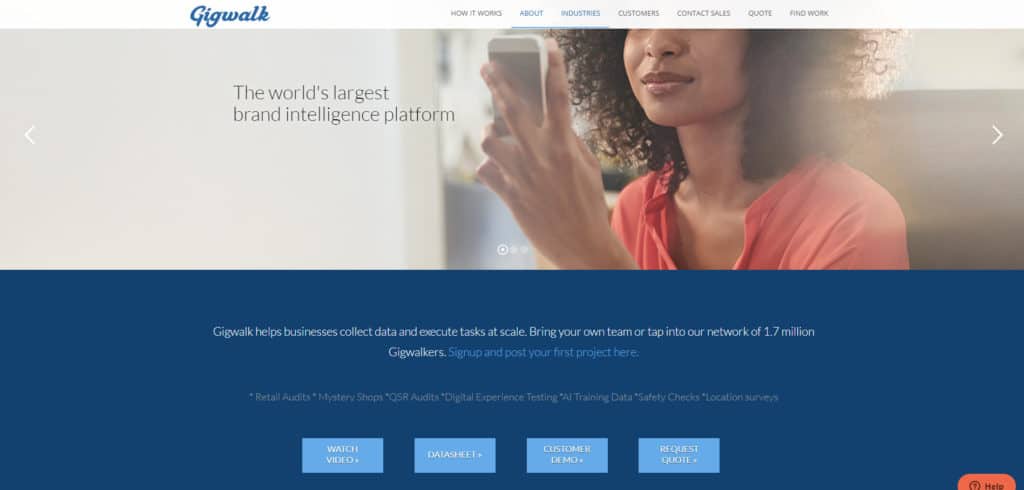The image depicts a detailed web page for Gigwalk, a brand intelligence platform. At the top of the page, "Gigwalk" is prominently displayed in blue letters. To the right, the navigation menu includes options such as "How It Works," "About," "Industries," "Customers," "Contact," "Sales Quote," "Find Work," and more. 

Central to the image is a photograph of a woman holding a white smartphone in her left hand, engrossed in its screen. Adjacent to her image, bold text proclaims, "The World's Largest Brand Intelligence Platform."

Below this, set against a darker blue background, lighter blue text outlines the platform’s features: "Gigwalk helps businesses collect data and execute tasks at scale. Bring your own team or tap into our network of 1.7 million gig walkers. Sign up and post your first project here."

Towards the lower section, four distinct rectangular buttons display options to "Watch Video," "Data Sheet," "Customer Demo," and "Request Quote." Above these buttons, in light blue text, various services offered by Gigwalk are listed, including "Retail Audits," "Mystery Shops," "QSR Audits," "Digital Experience Testing," "AI Training Data," "Safety Checks," and "Location Surveys."